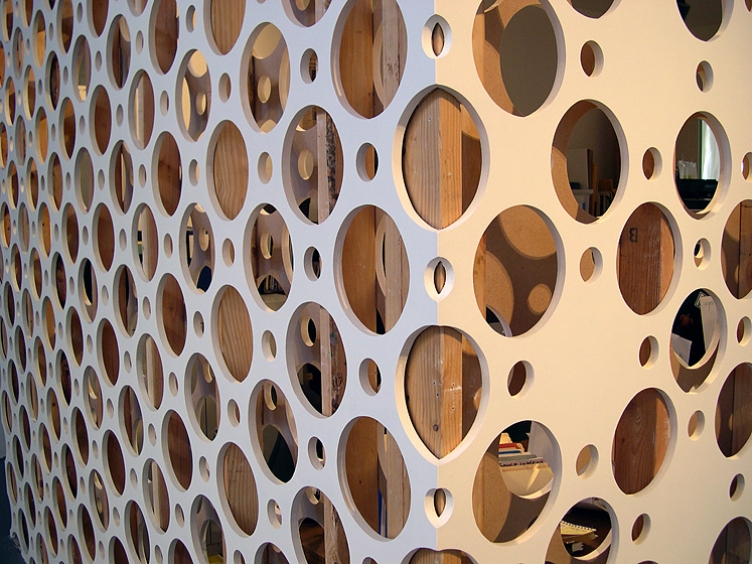This photograph captures what appears to be a corner section of a cubicle divider, featuring two white surfaces joined at a right angle. The surfaces are uniformly perforated with a combination of small and large circular holes, resembling the appearance of Swiss cheese. Through these symmetrically arranged holes, one can see wooden beams (likely 2x4s) providing structural support. Beyond the beams, the image reveals various office supplies and storage items, including a collection of files and papers in assorted colors such as red and blue, as well as a brown folder with black writing on its label tab. Additional visible items include a notebook, a disk, and in the top right corner, a shelf holding a board marked with the letter "B." This intricate composition suggests a glimpse into an organized, yet somewhat cluttered, storage area within an office environment.